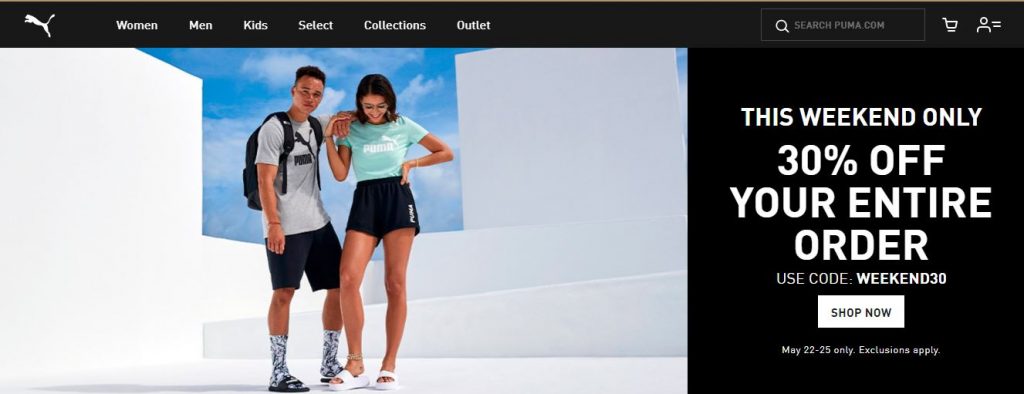The screenshot captures the homepage of the Puma website, featuring a black top navigation bar with a white Puma logo on the left side. The navigation bar includes several categories: Women, Men, Kids, Select, Collections, and Outlet. On the far right, there is a search bar labeled "searchpuma.com," followed by a shopping cart icon and an account button.

Dominating the center of the screen is a large promotional graphic set against a white background. The central image showcases a clear blue sky with scattered clouds. In the foreground, two models are prominently featured: a male on the left wearing a gray Puma shirt, a black backpack, black shorts, black and white socks, and black slides, and a female on his right with shoulder-length black hair, dressed in a teal Puma shirt, black Puma shorts, and white slides.

To their right, a black text box with white lettering announces a special weekend promotion: "This weekend only, 30% off your entire order. Use code WEEKEND30." Below this message is a "Shop Now" button. Further details indicate that the offer is valid from May 22 through May 25th, with exclusions applying.